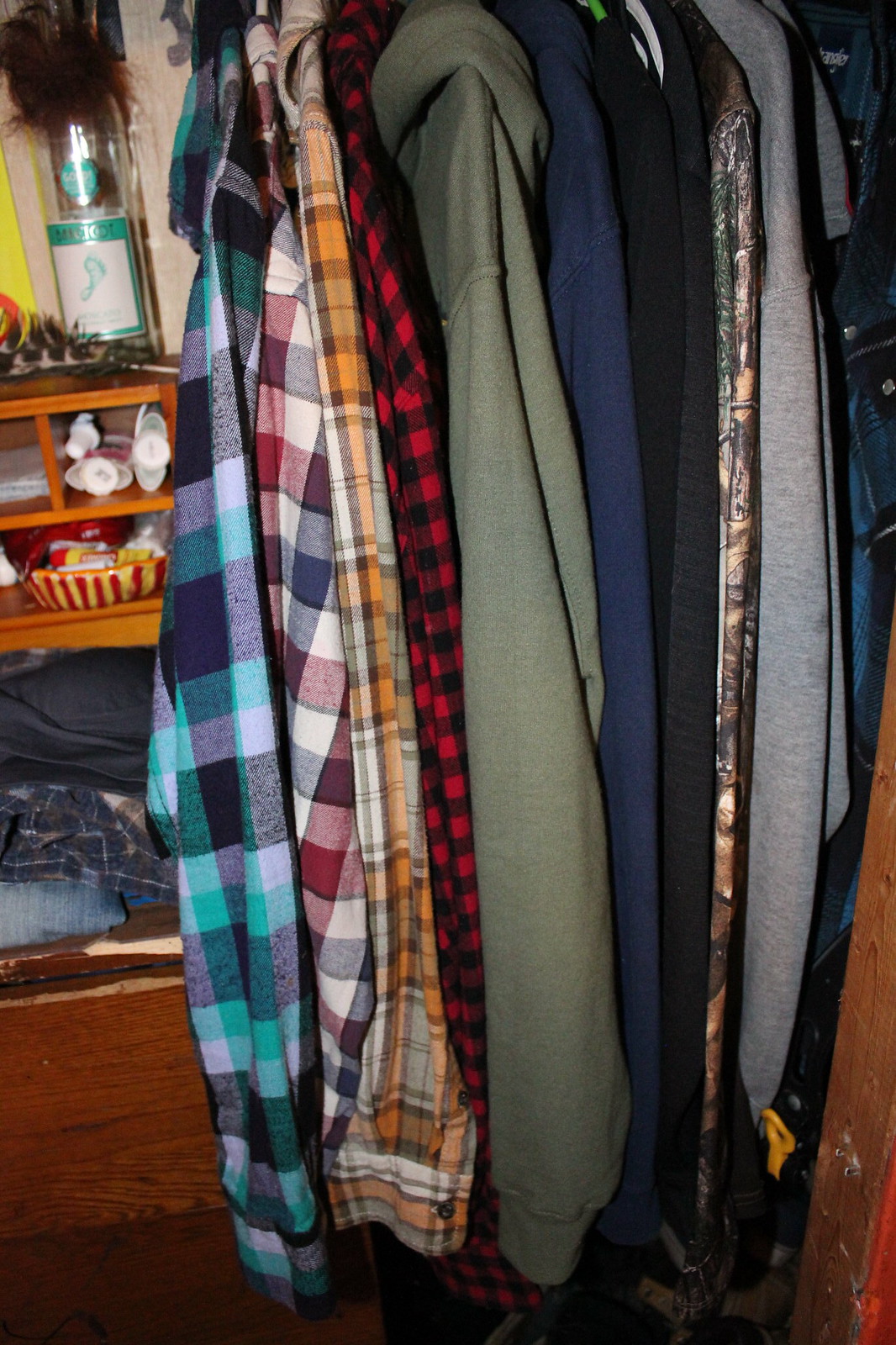This photograph captures the interior of a tall, narrow closet space. On the right-hand side, a diverse collection of at least ten shirts are hung neatly on hangers. The first few shirts are flannel button-downs, including a green and blue checkered one and a red, black, and white checkered one. Next, there are several hoodies, notably a green hooded sweatshirt and a blue sweatshirt, with additional shirts behind them, creating a visually dense array of clothes.

To the left, the back wall features a set of brown wooden shelves. The top shelf houses a bottle of wine, identifiable by its label which depicts a foot, suggesting it is from the Barefoot brand. Below this shelf, there is a partially visible one holding deodorant sticks. Further down, a small, vibrantly striped basket in shades of orangey-yellow and medium red sits on another shelf, containing various objects, possibly including Carmex. The shelves also display other toiletries like toothpaste. The depth and variety of items give this closet space a well-used, personal feel.